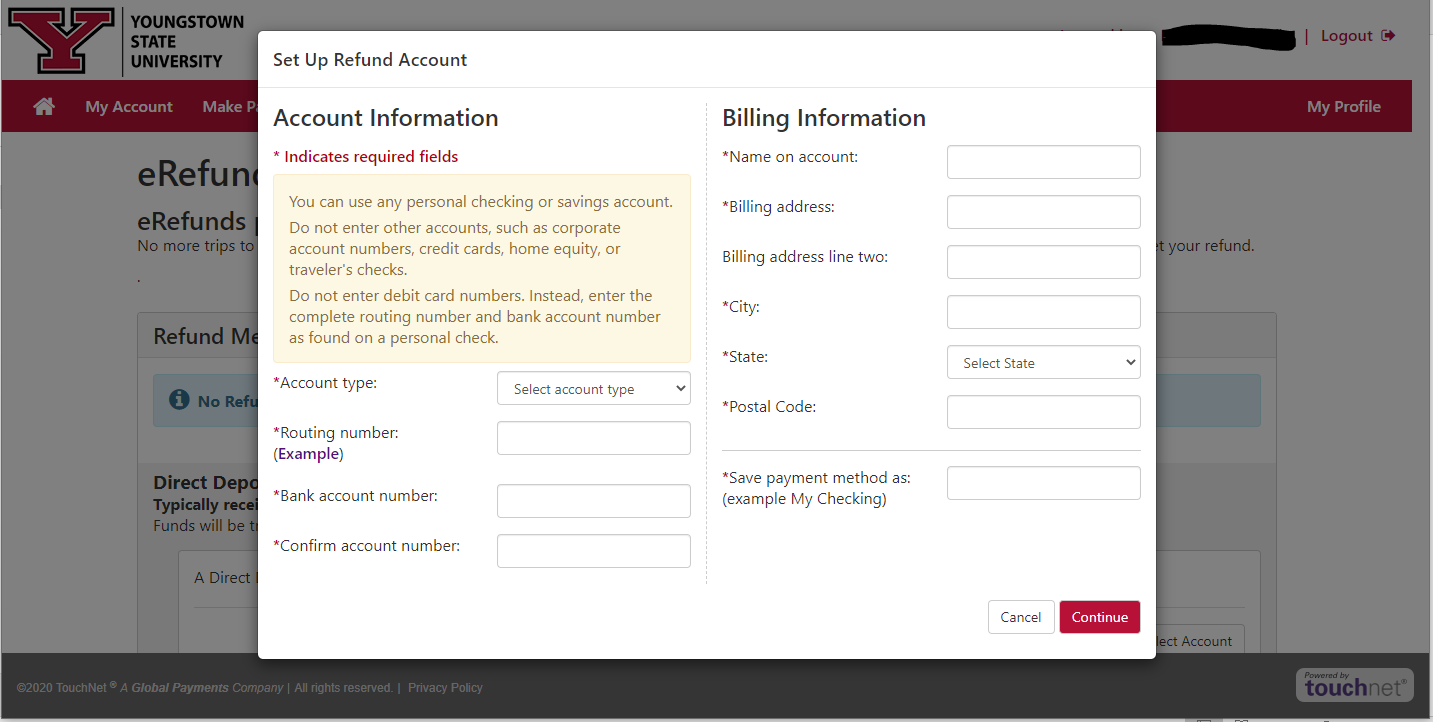In the foreground of the image, there is a white pop-out text box with black and red text on a webpage. The box is titled "Setup Refund Account" and provides fields for account information. Below the title, in smaller red text, it says "Indicates Required Fields." A prominent yellow box provides a detailed informational note, cautioning users to only enter personal checking or savings account numbers, emphasizing not to use corporate accounts, credit cards, home equity, travel checks, or debit card numbers. It instructs users to enter the complete routing number and bank account number as found on personal checks.

Directly underneath this yellow box are several fields to be filled out: "Account Type," "Routing Number," "Bank Account Number," and "Confirm Account Number." To the right of these fields is another section containing more boxes labeled "Billing Information," "Email Account," "Billing Address," "Billing Address Line 2," "City," "State," and "Postal Code." Beneath these fields, there’s an option to save the payment method, with an example provided ("my checking").

In the bottom right corner of the pop-out box, there are two buttons: "Cancel," which has a white background with black text, and "Continue," which also has a white background but with white text.

In the background of the image, the website for Youngstown State University is visible. In the upper left corner of the webpage, there is a large "Y" next to the words "Youngstown State." On the right side of the webpage, there is a logout icon, as well as some refund information.

Overall, the image shows a detailed and structured pop-out text box for setting up a refund account, superimposed over a webpage belonging to Youngstown State University.